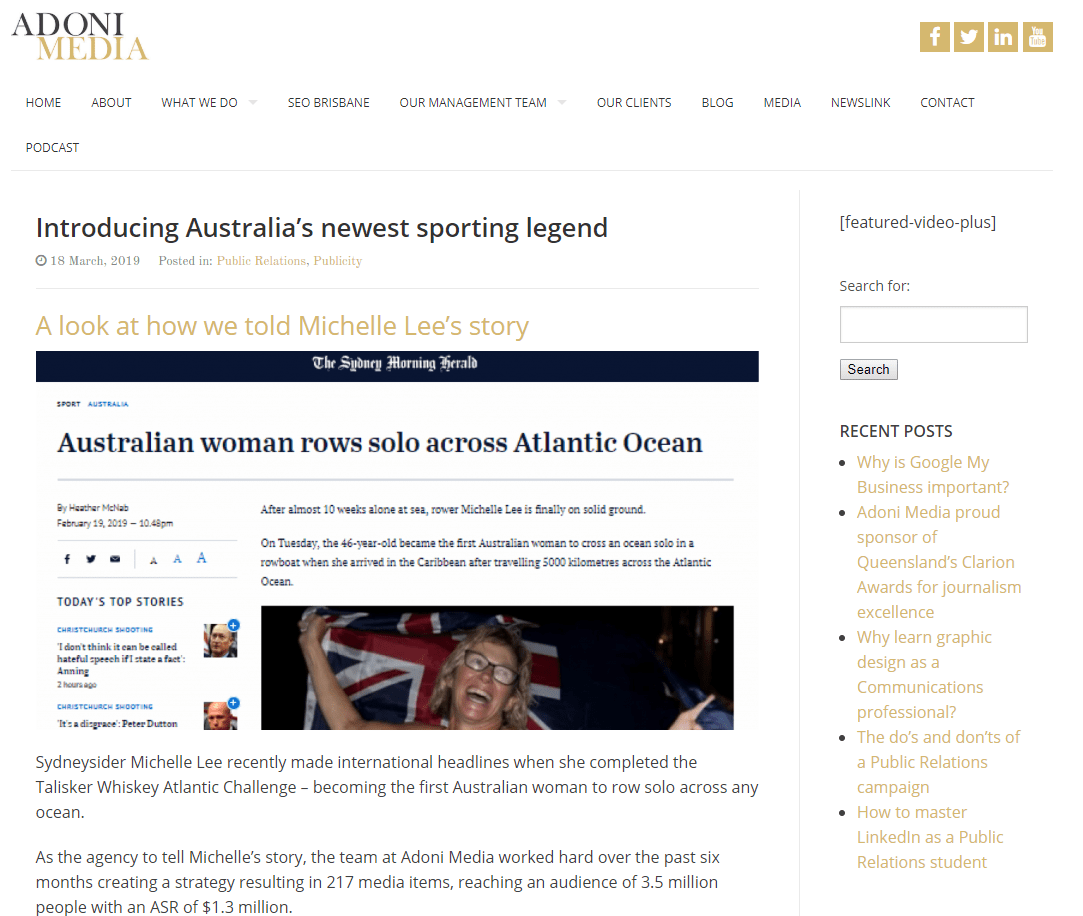O'Donnie Media's homepage prominently displays their name, with navigation links for sections such as "Home," "About," "What We Do," "SEO Brisbane," "Our Management Team," "Our Clients," "Blog," "Media," "News Link," "Contact," and "Podcast." 

The highlight of the page is a feature story introducing Australia's newest sporting legend, Michelle Lee. The headline narrates the remarkable achievement of Michelle Lee, who became the first Australian woman to row solo across the Atlantic Ocean. The detailed account reveals that after nearly 10 weeks alone at sea, Lee successfully completed her journey, covering 5,000 kilometers and arriving in the Caribbean. 

O'Donnie Media prides itself on being the agency responsible for sharing Michelle Lee's extraordinary story. Over the past six months, their strategic efforts culminated in the creation of 217 media items, which reached an impressive audience of 3.5 million people, generating an ASR (Advertising Space Rate) of $1.3 million. The feature underscores the agency's capability in effective storytelling and media strategy.

Additional context is provided about Michelle Lee's feat, noting that she garnered international attention when she completed the Talisker Whisky Atlantic Challenge. Particularly, the story was highlighted by a prominent feature in the Sydney Morning Herald, recognizing Michelle Lee's incredible perseverance and monumental accomplishment.